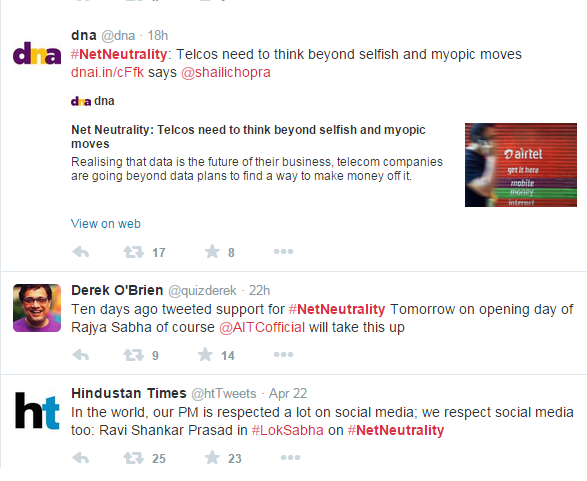The image features a white background with several Twitter posts. The top tweet is from a user with the handle @DNA, and their profile picture showcases the letters "DNA" with the 'D' and 'A' in purple, while the 'N' is yellow. The tweet was posted 18 hours ago and includes the hashtag #NetNeutrality. The content of the tweet reads: "Telcos need to think beyond selfish and myopic views. Realizing that data is the future of their business. DNA.in/cffk mentions @chalet hopro. Telcos are going beyond data plans to find a way to monetize it."

Below the tweet, there is a blue hyperlink labeled "View on web," indicating that the tweet can be viewed online. The tweet has received 17 shares and 8 likes.

The second tweet in the image is from Derrick O'Brien, using the handle @QuidDerrick. This tweet was posted 22 hours ago and references a tweet from 10 days prior. It reads: "Support for net neutrality tomorrow on the opening day of Rajya Sabha. Of course, @AITCOfficial will take this up."